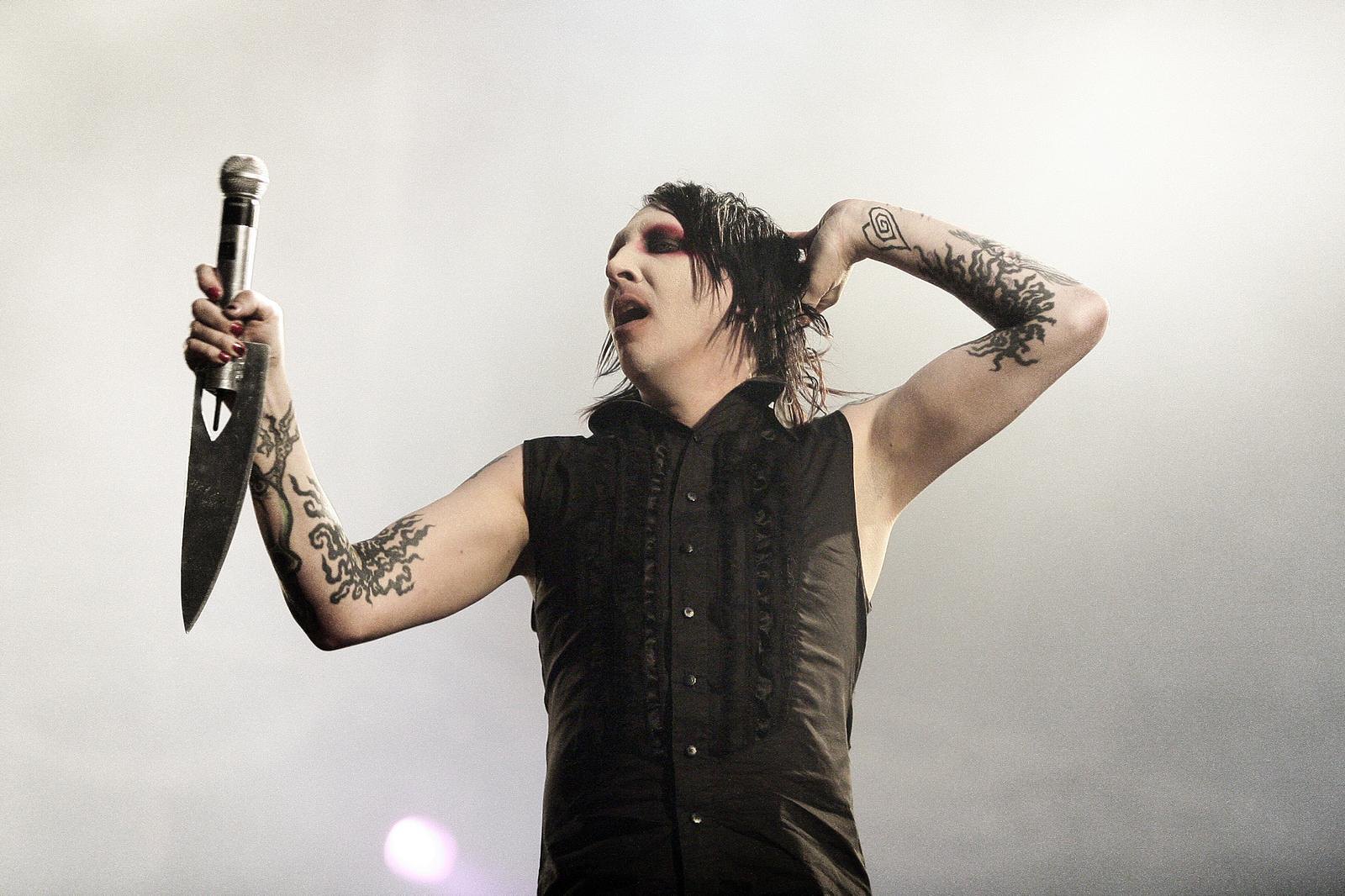In an off-white, out-of-focus background that hints at stage lights, a person channels the intense style of a heavy metal rock star. With greasy, disheveled black hair, their head tilts slightly to the left as they face the camera with a dramatic flair. Their left arm is raised and resting behind their head, while their right arm, adorned with tattoos, including a heart and various lines, grips a large, ancient-looking dagger that evokes medieval times. They sport a high-collared, sleeveless black shirt fastened with silver buttons, and their nails are painted. The person's eyes are strikingly painted black and reddish, adding to their theatrical appearance.